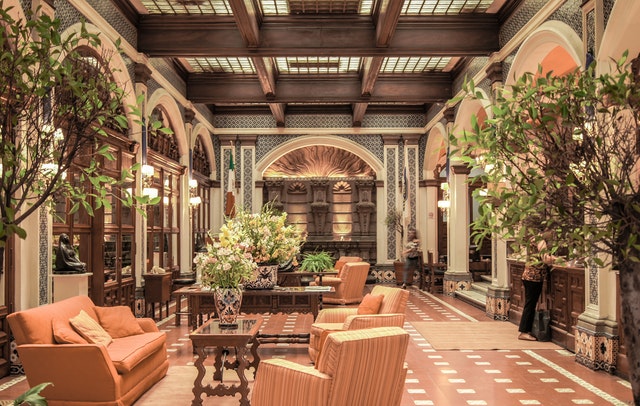The image depicts a luxurious and expansive hotel lobby, characterized by its ornate and meticulous design. The high ceiling features exposed brown beams traversing the space, interspersed with glowing white grids that lend an airy, skylight effect. The room is decorated with large, elegant arches, each framed in white with intricate mosaic bases and further detailed in dark brown wood.

Flanking the room to the left and right are indoor trees, adding a natural touch to the sophisticated ambiance. Warm orange couches encircle a central glass coffee table adorned with an ornate vase brimming with flowers. Directly behind this seating area sits a larger table, also lavishly decorated with an expansive floral arrangement.

The back wall is lined with shelves, highlighted by striking blue and white mosaics, and features a decorative arch that evokes an elaborate art piece. A combination of orange and white square tiles covers the floor, complemented by a large rug. A woman is seen in the background, partially obscured by the interior foliage.

On the right side of the image, likely the check-in area, another woman stands beside a counter with luggage, underscoring the space’s function as a hotel lobby. The use of exposed wooden beams, broad archways, and glass-topped tables with floral vases creates a welcoming yet opulent environment, perfect for a hotel of this caliber.